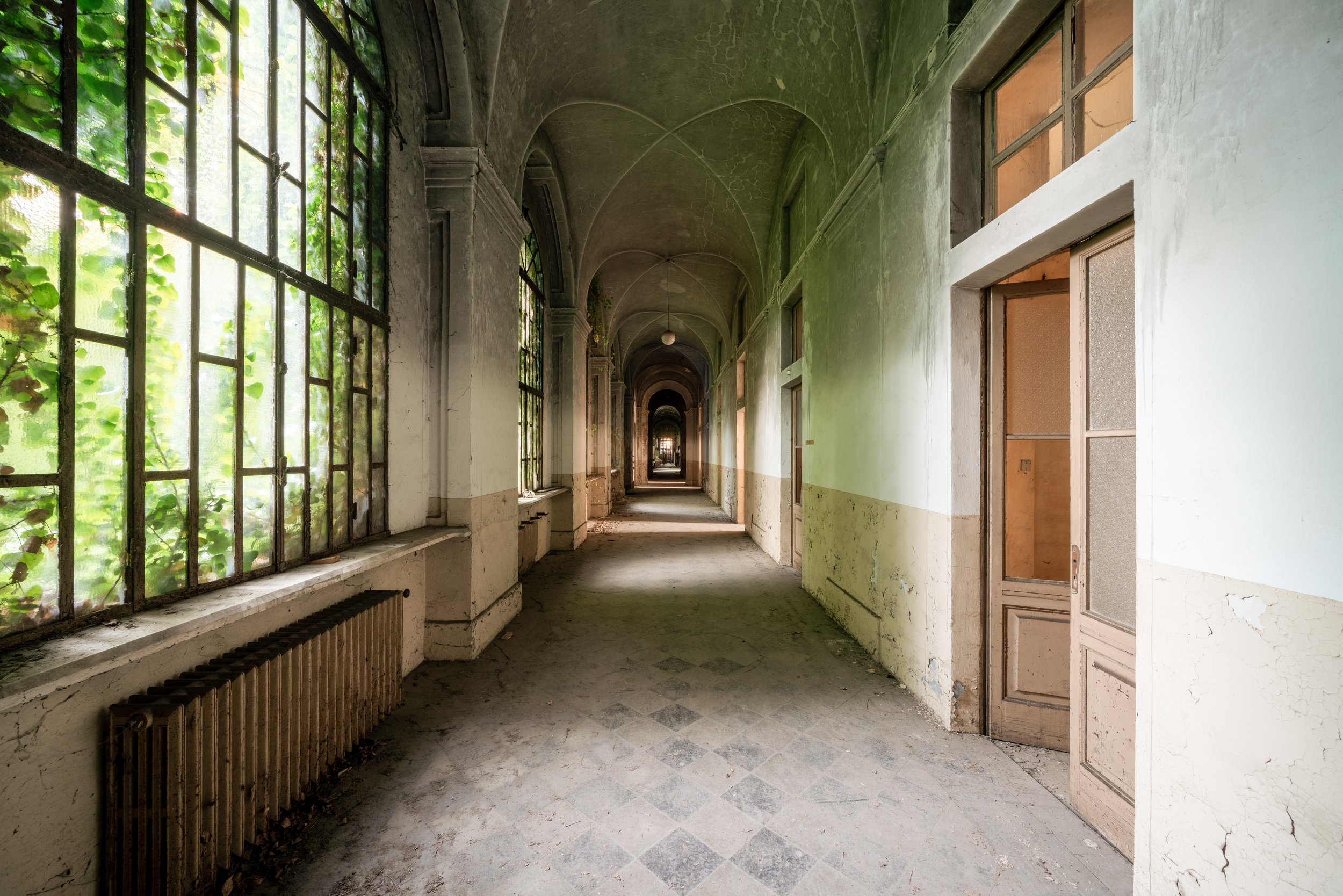This photograph captures a long, narrow interior hallway within an abandoned building. The hallway is centrally framed within the nearly square photograph, extending deeply into the background. The wall surfaces, originally white, show significant wear with peeling wallpaper and paint, transitioning into shades of green and dark gray higher up. The flooring, once presumably white, has dulled to a dirty gray. A row of windows lines the left side, densely covered with pressing leaves, suggesting an overgrown exterior environment. A radiator is also visible on this side. On the right, there are double wooden doors painted white, set beneath a large window, some glass panes of which are shattered or missing. The ceiling is similarly deteriorated, though a lone hanging light fixture remains intact but unlit. The hallway is characterized by a series of arches, culminating in multiple archways that provide a view into another room further behind. The overall color palette of the image includes muted browns, tans, whites, grays, greens, and blacks, emphasizing the decrepit state of the building in broad daylight.